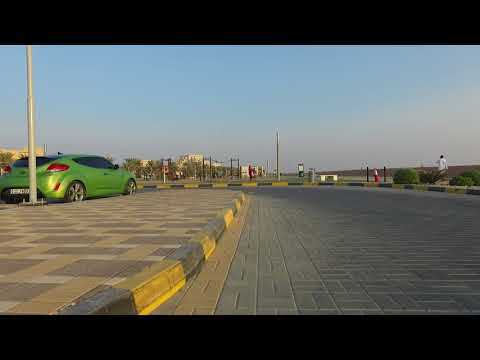The image is a color photograph, landscape-oriented, capturing an outdoor scene with a clear blue sky, transitioning to a purplish hue near the horizon, suggesting it was taken at or near sunset. The ground is evenly flat, adorned with a gray cobblestone pattern. On the left side of the photo, there is a vibrant green sporty two-door sedan, potentially of European make, parked near a large silver pole. Adjacent to the vehicle is a concrete island painted with a yellow and black checkerboard pattern. In the right foreground, a person in a white shirt can be seen walking along a pathway. Further back, commercial buildings and sections of green vegetation dot the landscape, with several poles scattered throughout. The overall color palette includes blue, yellow, black, gray, green, red, and white hues, contributing to the photographic realism of the scene. The area resembles a parking lot or a space near a park, devoid of clouds and filled with various details that bring the image to life.